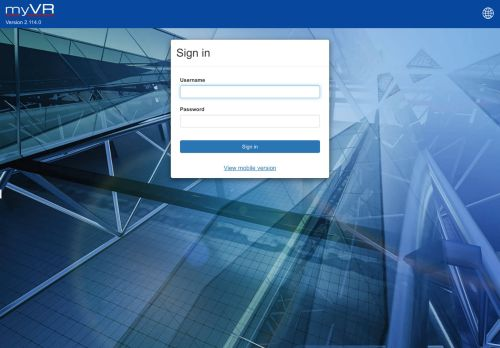A window with a "sign in" prompt takes center stage in this vibrant VR interface, displaying version 2.11.4.0. The screen shows a blue bar at the top, adjacent to a white bar where users can input their username and password. Below, a blue rectangle with the text "Sign In" stands out, accompanied by an option to view the mobile version. The background is an intricate architectural design, featuring crisscrossing metal bars and a grid of glass squares against a clear blue sky. This fascinating combination of structure and technology presents a visually engaging scene.